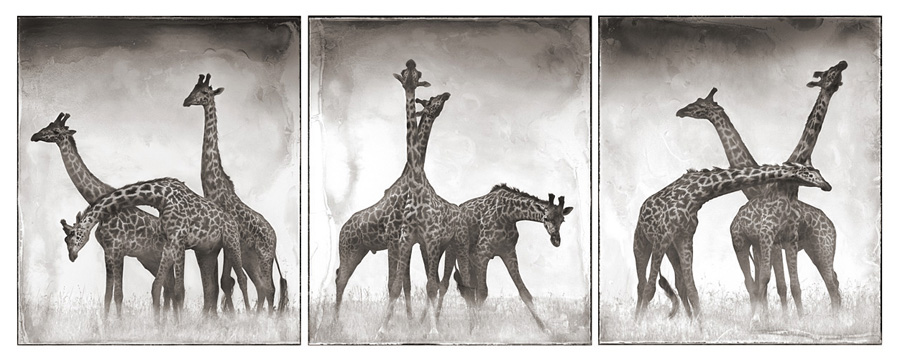This is a composite artwork consisting of three contiguous black-and-white images, each depicting three giraffes in various poses. The images are arranged side-by-side, forming a cohesive art collection. In the left image, all three giraffes are gazing to the left; two have their heads held high while one has its head lowered toward the ground. The middle image portrays three giraffes with two of them intertwining their necks and looking up at the sky, while the third giraffe directs its head downward and to the right. The rightmost image again includes three giraffes, one looking left, one looking right, and another with its neck stretching upward towards the upper right. Each image is set against a simple backdrop, featuring a white background with subtle black smudges, giving a sense of texture and depth. The giraffes are standing in a tall, overgrown field, creating an interconnected and dynamic visual narrative.